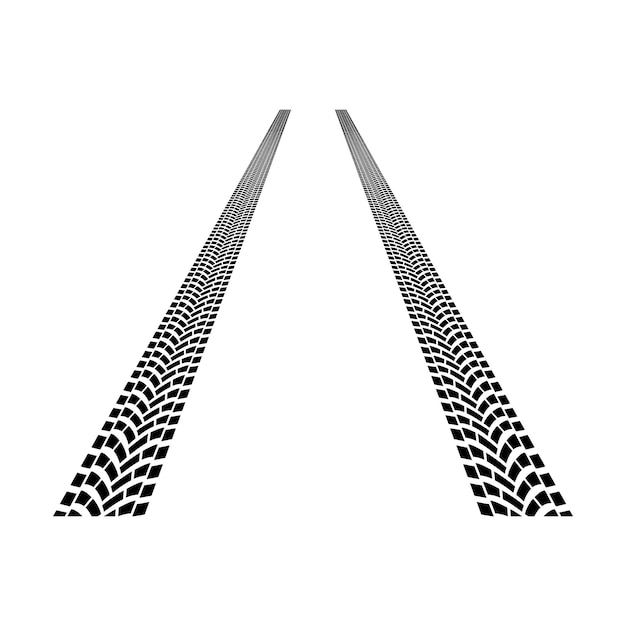The graphic design depicts two elongated black tire tracks on a pure white background, resembling the remnants of a vehicle driving away from the viewer. The tracks are initially thick and detailed in the foreground, showcasing a repeated pattern of dashed rectangular lines on the sides and curvy rectangular lines drooping downward in the center. As the tracks recede into the background, they get narrower and blurrier, converging slightly towards the middle of the image at the top. The distance between the tracks suggests they are from a car or truck, and the design features six distinct points of contact on each tread, running continuously for what appears to be at least 100 feet.